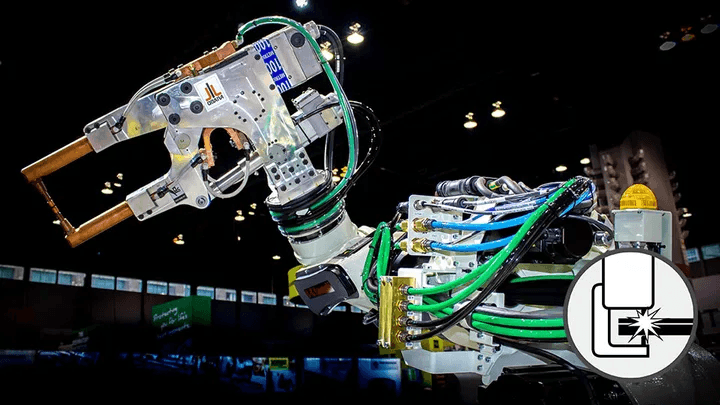The image depicts a large, silver, pneumatic-controlled robot arm with various green, blue, and black hoses intricately connected to it. The arm features orange prong-like hooks near its end, along with visible black screws. At the top, there's a blue label, and a notable element is an orange component with a silver tip connected to a green hose, which wraps around the base. The central machinery feeds into another piece of equipment, with the hoses securely fastened to it. An illustrative black-and-white sketch in the bottom right corner, possibly detailing a part of the robot, shows a section resembling a fuse box with a star-like depiction that may suggest a flame or spark. The scene is set against a dark background, likely inside a warehouse or industrial building, evidenced by visible overhead lights and additional machinery. A silver metal box with a yellow glass light, which could be illuminated when powered on, is also part of the setup.